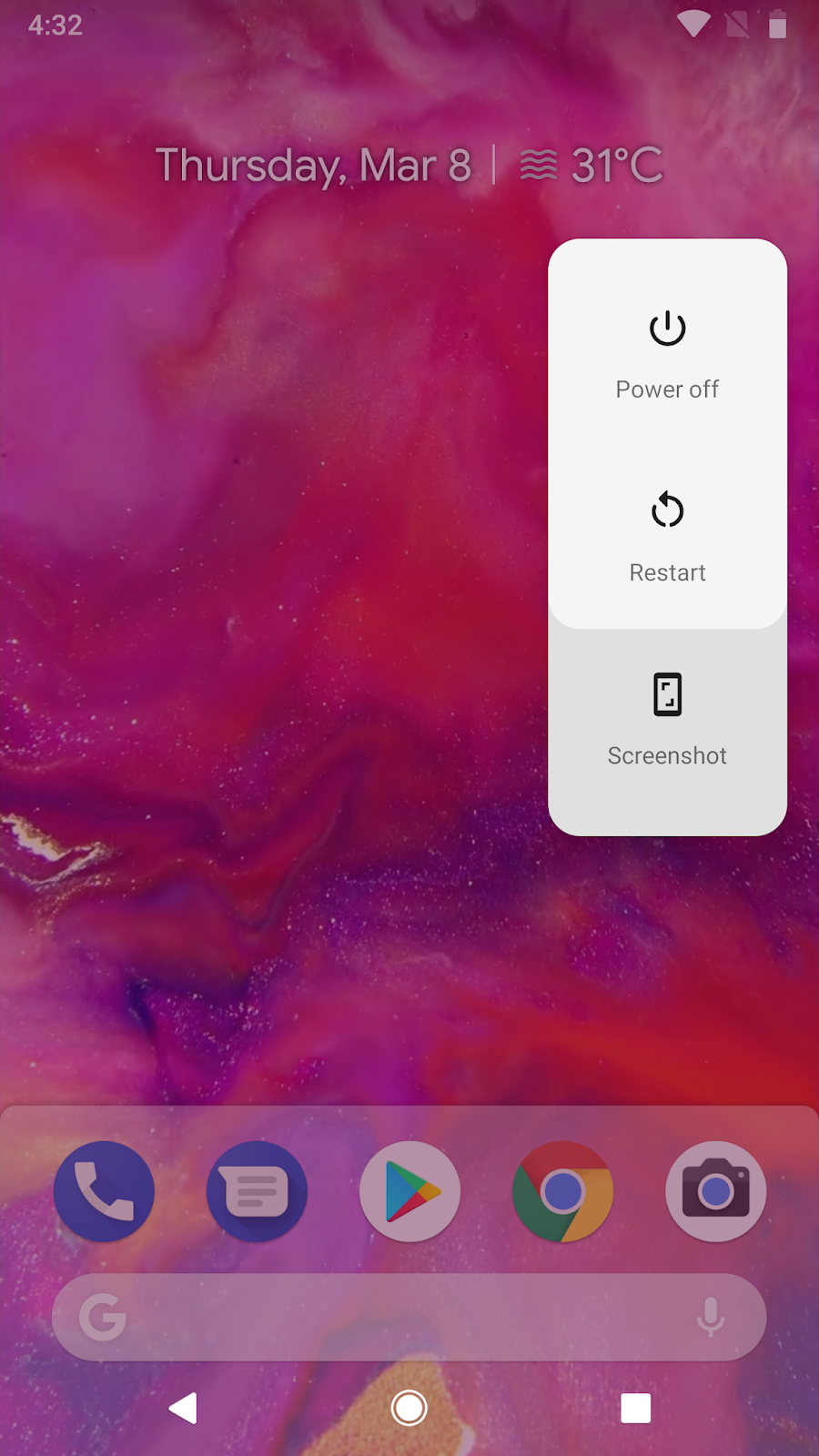The Android homepage showcases a striking purple background, intricately infused with swirls of red, creating a mesmerizing marbled pattern. Adhering to a minimalist design, the top of the screen displays the current date, Thursday, March 8th, with a weather icon indicating fog and a temperature of 31°C, suggesting warm conditions. Positioned towards the middle right, a floating menu action bar provides quick options for power off, restart, and screenshot, likely accessed by long-pressing the power button. The screen is nearly icon-free except for a bottom row that remains consistent across different screens, featuring essential apps: Phone, Messages, Google Play, Chrome, and Camera. Below these icons is a gray search box adorned with a 'G' on the left and a microphone icon on the right. At the very bottom, indicative of an older Android version, are the familiar navigation buttons: Back, Home, and App List.